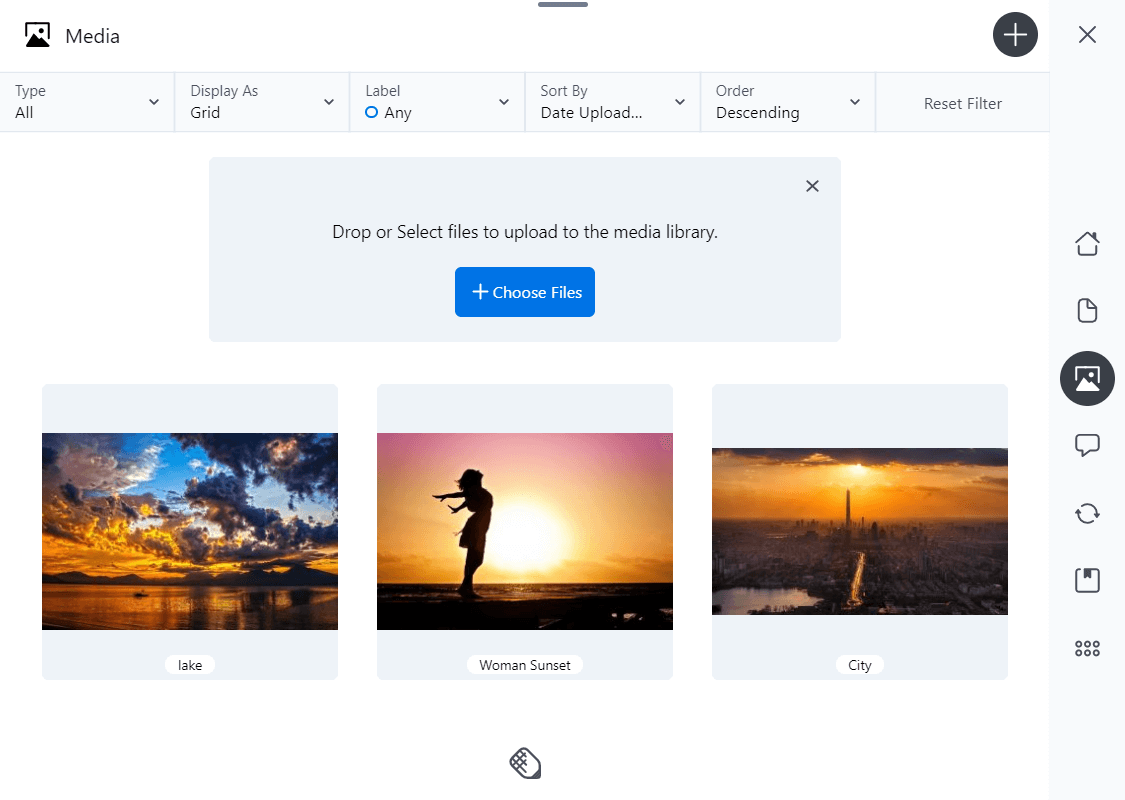This screenshot image features a media management interface. At the very top left corner, there is the word "Media." Below it, a series of tabs are visible. The first tab reads "Type: All" accompanied by a drop-down arrow. Following it is a tab labeled "Display as: Grid," also with a drop-down arrow. The next tab, marked with a blue circle, reads "Label: Any" and has its own drop-down arrow. Continuing along the line, the tab "Sort by: Date Uploaded" can be seen, again with a drop-down arrow. The subsequent tab lists "Order: Descending," paired with a drop-down arrow, and finally, there is a "Reset Filter" tab.

Beneath these tabs, centrally located on the screen, there's a light-colored box. The box contains the instruction, "Drop or select files to upload to the media library." Below this message, there is a blue banner with a plus sign and the text "Choose Files." In the upper right-hand corner of this box, a small black 'X' is visible, presumably to close the box.

Dropping further down on the interface, three images are displayed side-by-side. The first image shows a serene lake, the second depicts a woman set against a breathtaking sunset background, and the third image captures a sprawling cityscape.